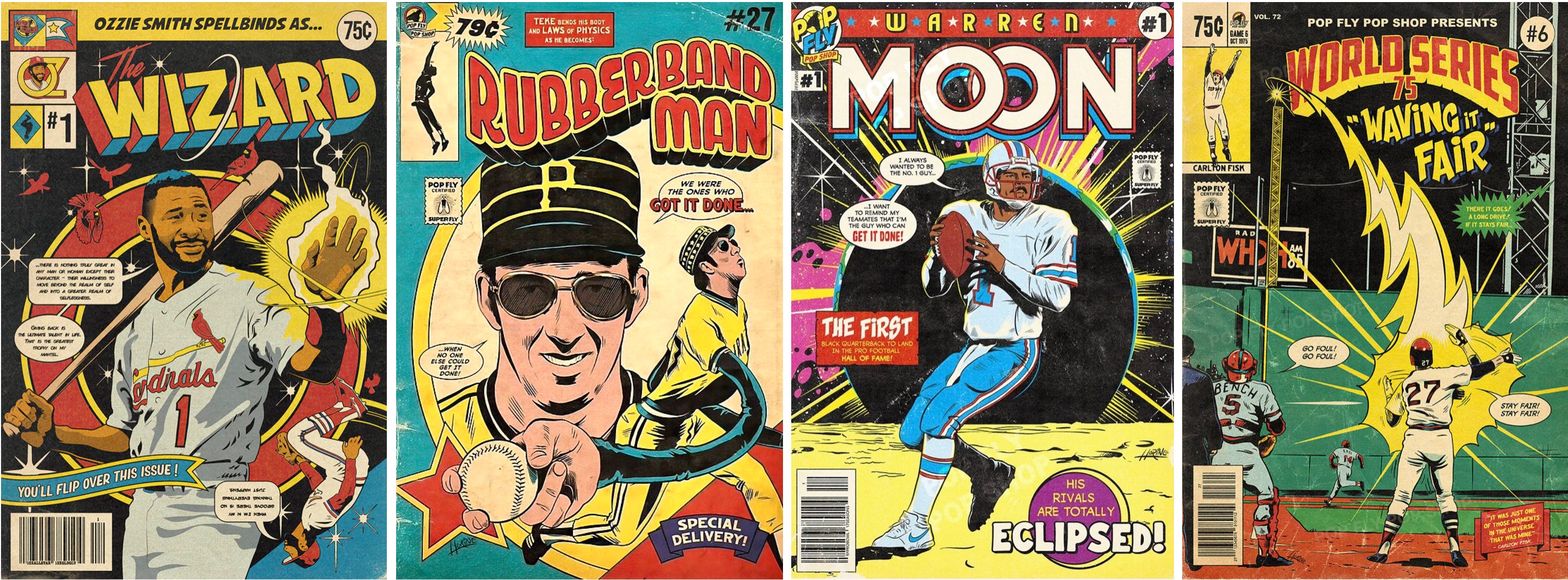This image showcases four distinct vintage comic book covers arranged in a row from left to right. The first cover features Ozzie Smith, depicted as a superhero with a glowing yellow hand under the title "Spellbinds as Wizard." The Cardinals player is adorned in a white Cardinals jersey, complete with facial hair and blue hair, holding a bat on his shoulder and extending his hand as if to wave or cast a spell. The second comic book, titled "Rubberband Man," portrays a man in a yellow outfit, pitching a baseball with his right hand, suggesting an incredible ability to stretch his limbs. The third book is titled "Moon," highlighting an NFL quarterback poised to throw a pass, donning a white jersey and blue football pants. Lastly, the fourth cover, marked with the title "World Series," features an intense depiction of a baseball player in a red jersey with the number 27. The player is framed by a dramatic thunderbolt and appears to either be pitching or catching a ball. All four covers represent a blend of sports heroes and fantastical elements, emphasizing baseball in three and football in one.